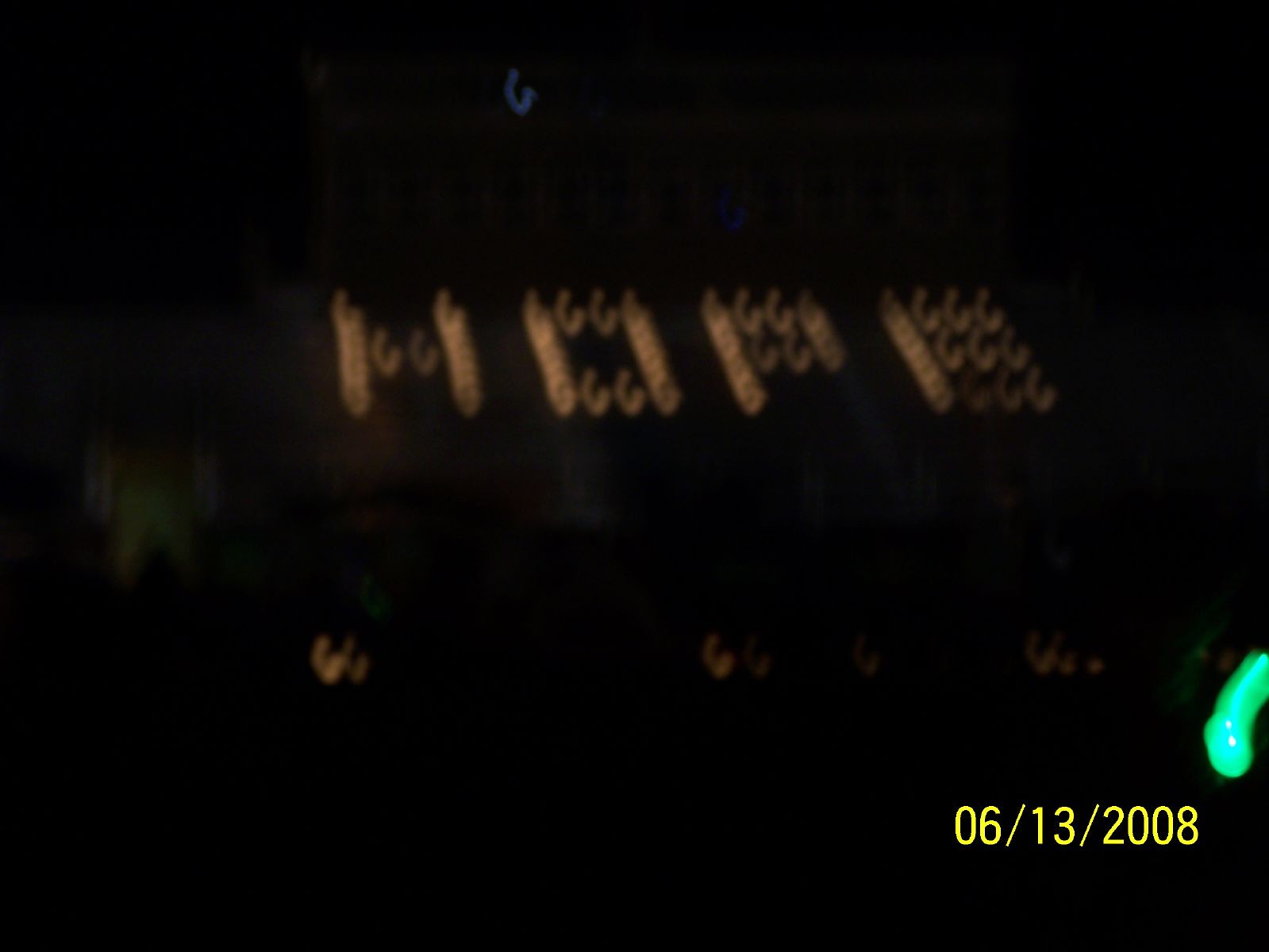This photograph, dated June 13, 2008, as noted in the bottom right corner, captures the word "HOPE" spelled out in lights against a predominantly dark background. The image appears to have been taken at night, contributing to its overall blurriness. The letters forming "HOPE" are whitish, with a light brown tint, arranged in a circular, spiral-like pattern, and occupy the upper middle portion of the frame, roughly the top 25%. Below these illuminated letters, scattered additional lights can be seen. Adding to the enigmatic scene, a green streak of light is visible just above the date in the lower right corner. The setting could be an outdoor location, possibly a stadium or some flat, slanted area, although the exact details remain unclear due to the image's blurriness.